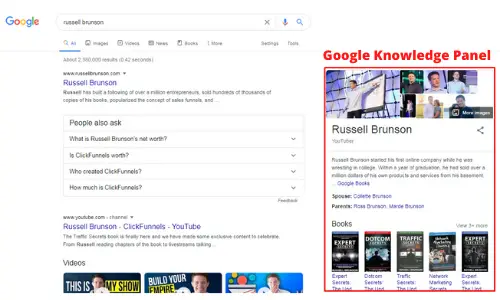The image depicts a Google search results page with a predominantly white background. At the top left corner, the well-known colorful "Google" logo is prominently displayed. Adjacent to the logo on the right is the search bar, which contains text that is too small and blurry to read clearly. On the far right of the search bar are three icons: from left to right, a gray "X," a microphone symbol, and a magnifying glass icon. Directly below the search bar, the navigation options are visible, with "All" underlined in blue, followed by "Images" and another indistinguishable option, all part of Google's typical layout.

In the main body of the search results, the name "Russell Burson" appears in purple text, indicating it is a clicked or visited link, with additional information listed beneath it. At the bottom of the page, there is a section labeled "Videos," where the upper portions of three clickable video thumbnails are displayed. Each thumbnail features a blue background: the left and middle thumbnails have a dark blue hue, while the rightmost one is a lighter blue.

On the right side of the page, there is a designated area titled "Google Knowledge Panel," highlighted in red lettering. Below this title is a red-outlined box containing the name "Russell Brunson" along with a substantial amount of text. Also displayed within this box are images of various books, each featuring a predominantly dark black cover.